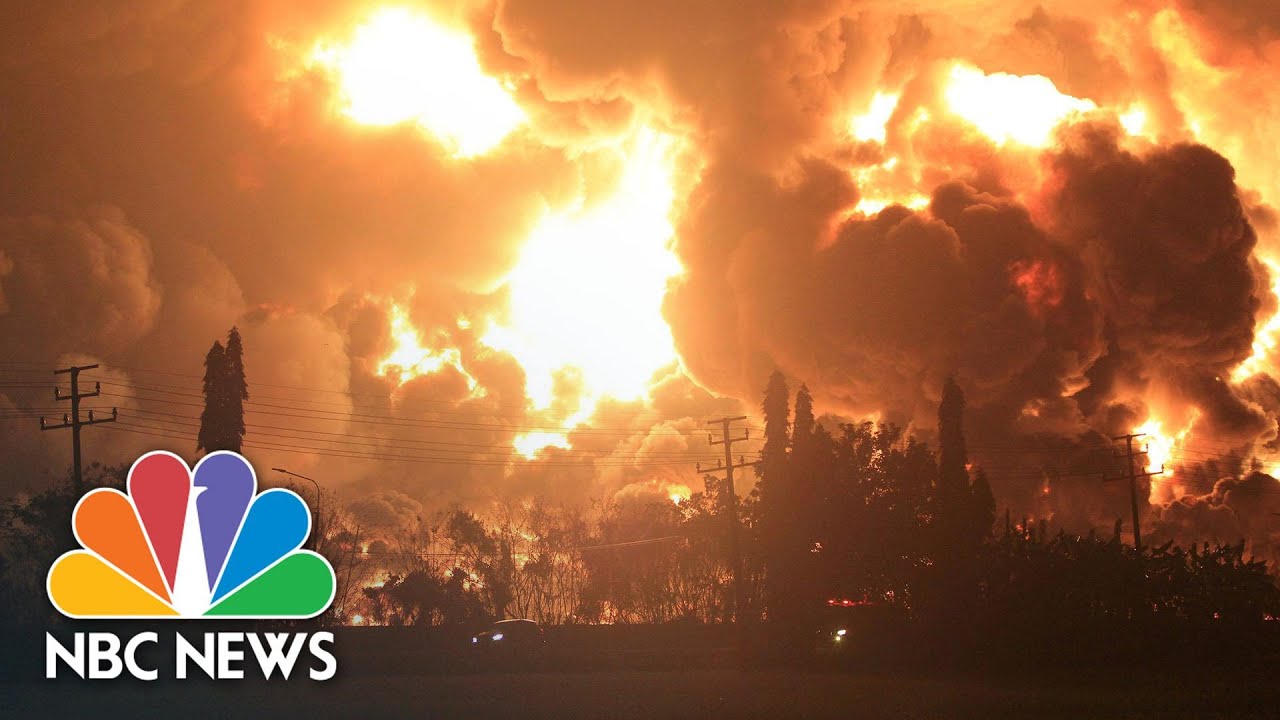A widescreen photo, credited to NBC News with the distinctive peacock logo on the lower left, captures a dramatic nighttime scene dominated by a massive, blazing fire. The sky is a fiercely lit tapestry of bright orange and yellow, smothered with dark, billowing clouds of smoke that give the image an ominous, apocalyptic feel. Silhouetted trees and power lines stretch across the foreground, their outlines stark against the fiery sky. At the bottom of the image, several vehicles with visible headlights move from right to left, their presence barely discernible in the low light, adding to the sense of urgency and chaos. This striking image, with its vivid colors and stark contrasts, conveys a sense of impending disaster.